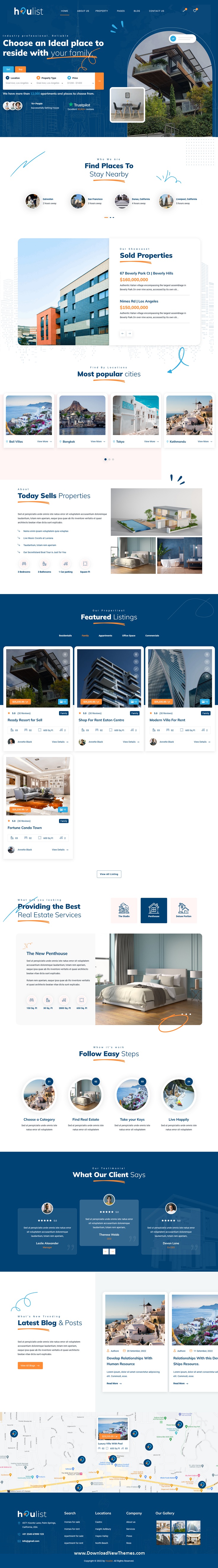This is a detailed caption for the image based on your description:

"This is a smartphone screenshot of a web page, likely focused on affordable residential or lodging options. The page prominently features the phrase 'cheaper' in relation to an ideal place to reside. The layout includes various images of structures, both exterior and interior, which appear to be a mix of apartment buildings, corporate buildings, and possibly hotels. At the top of the page, there are images that likely depict corporate buildings. Scrolling down, the page shows photos of rooms, including one with a bed next to a window, hardwood floors, and bedside lamps, suggesting it could be a hotel room. The bottom of the page features a section titled 'What Our Clients' and includes exterior photographs as well as a Google map snippet. The images are mostly taken during the daytime, though some are captured in the evening. One of the interior photos clearly shows a bedroom, further supporting the idea that these are accommodations for living or staying temporarily."